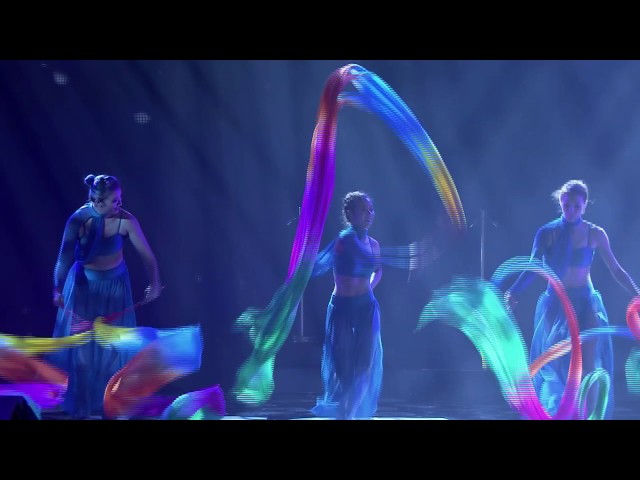This image is a landscape-oriented, color photograph that captures a freeze-frame from a video, most likely from a televised performance. It features three women standing side-by-side against a dark blue backdrop, each performing a ribbon dance. The three women, dressed in matching dark blue halter tops and long, silky, see-through pajama-like skirts, evoke an exotic, Aladdin-esque style. Their outfits reveal their midriffs, adding a touch of allure to their coordinated dance movements.

The central performer is notable for her joyful expression, facing the right side of the image while twirling her multi-colored ribbon—comprising hues of yellow, blue, red, purple, and green—above her head in an arc. The two other dancers, positioned on the left and right, mirror her outfit and hairstyle, with their hair elegantly styled and packed. They both engage in ribbon twirling, creating mesmerizing spiral patterns with their colorful ribbons closer to the ground in front of them.

The photo has a pixelated quality, consistent with a video still, and is framed by horizontal black rectangles at the top and bottom, adding to the sense that this is a moment paused in time from an engaging live performance.